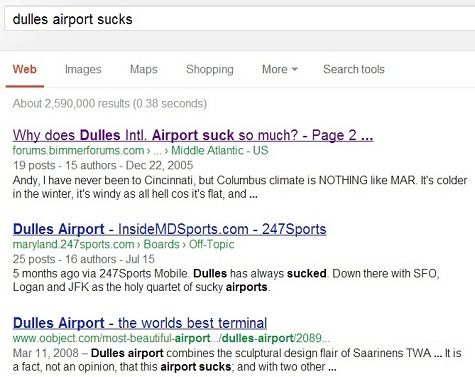In the image, a web search page is displayed with an individual expressing frustration about Dulles International Airport. The search bar at the top prominently features the query "Dulles Airport sucks," highlighting their dissatisfaction. Below the search bar, various search options such as Web, Images, Maps, Shopping, More, and Search Tools are visible. The search yields nearly 2.6 million results. 

The leading result is titled "Why does Dulles International Airport suck so much?" from the forums on Bimmer forums, dated December 22, 2005. It consists of 19 posts from 15 different authors, with one user expressing that while they have never been to Cincinnati, the colder, windier climate of Columbus is comparable to Dulles, though the relevance to Dulles is unclear.

The second result from mdsports.com, dated five months ago and featuring 25 posts from 16 authors, maintains the negative sentiment. It compares Dulles unfavorably to other notorious airports like SFQ, SFO, Logan, and JFK, labeling them collectively as the "holy quartet of sucky airports."

Contrastingly, the third result carries a more positive tone. Titled "Dulles Airport, world's best terminal," it suggests that not all users share the negative perspective, indicating a mix of reviews.